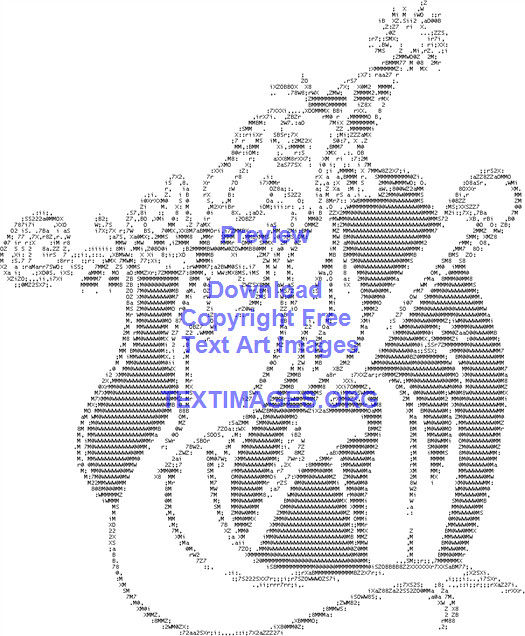This black-and-white, grainy digital graphic features an older man depicted as a wizard. He has a long beard that reaches the floor and is dressed in robes. On his head, he wears a cone-shaped hat, which features a circular design and is topped with a white pom-pom. The wizard holds a long rod in one hand, possibly a wand, and a birthday whistle or pipe in the other. The entire image is pixelated, rendered in white and gray squares or numbers, contributing to its text art style. Overlaid prominently in blue and purple text are the words: "Preview. Download copyright-free text art images. Textimages.org."